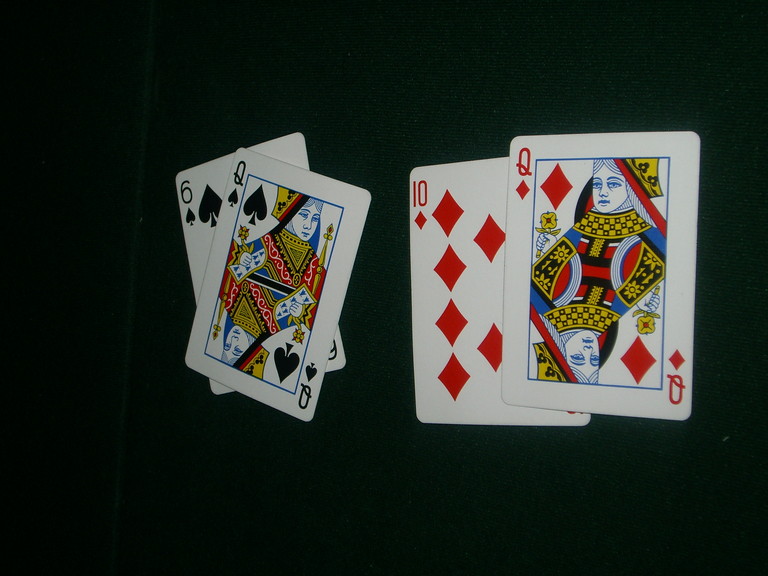In this photograph, four playing cards from a deck are meticulously arranged on a dark green poker table. On the right side, the red Queen of Diamonds is partially covering the red 10 of Diamonds, with only the bottom half of the 10 of Diamonds visible. To the left, the black Queen of Spades is positioned slightly askew, revealing the black 6 of Spades underneath. The top left corner of the Queen of Spades is turned inward, creating small visible slivers of the 6 of Spades in both the upper left and upper right corners. The arrangement highlights the contrasting colors and values of the cards against the rich green background of the poker table, suggesting a moment captured during a card game.